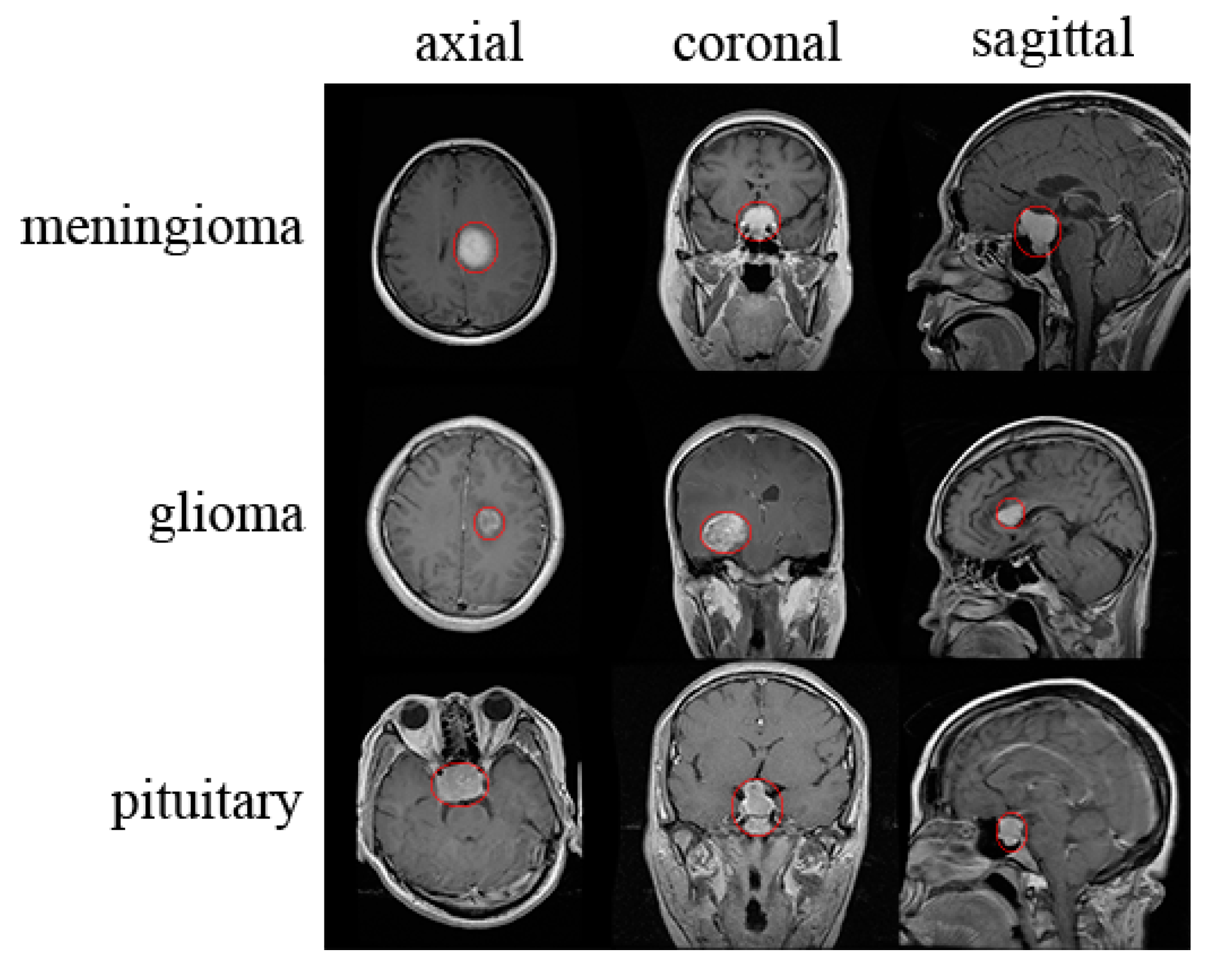The image is a 3x3 grid of nine detailed brain scans, presented against a black background and divided into rows and columns. The rows, labeled on the left side with "Meningioma," "Glioma," and "Pituitary," depict different types of brain conditions. The columns at the top are labeled "Axial," "Coronal," and "Sagittal," representing the top-down, back, and side views of the brain, respectively. Each grayscale scan has a distinct area highlighted with a red circle, indicating points of interest within the brain. The scans show various perspectives: the first column presents a top point of view, the middle column shows views from the back, and the right column displays side perspectives. Notably, features such as the eye sockets and specific brain regions are distinctly highlighted, providing a comprehensive visual comparison of the brain conditions across different anatomical planes.